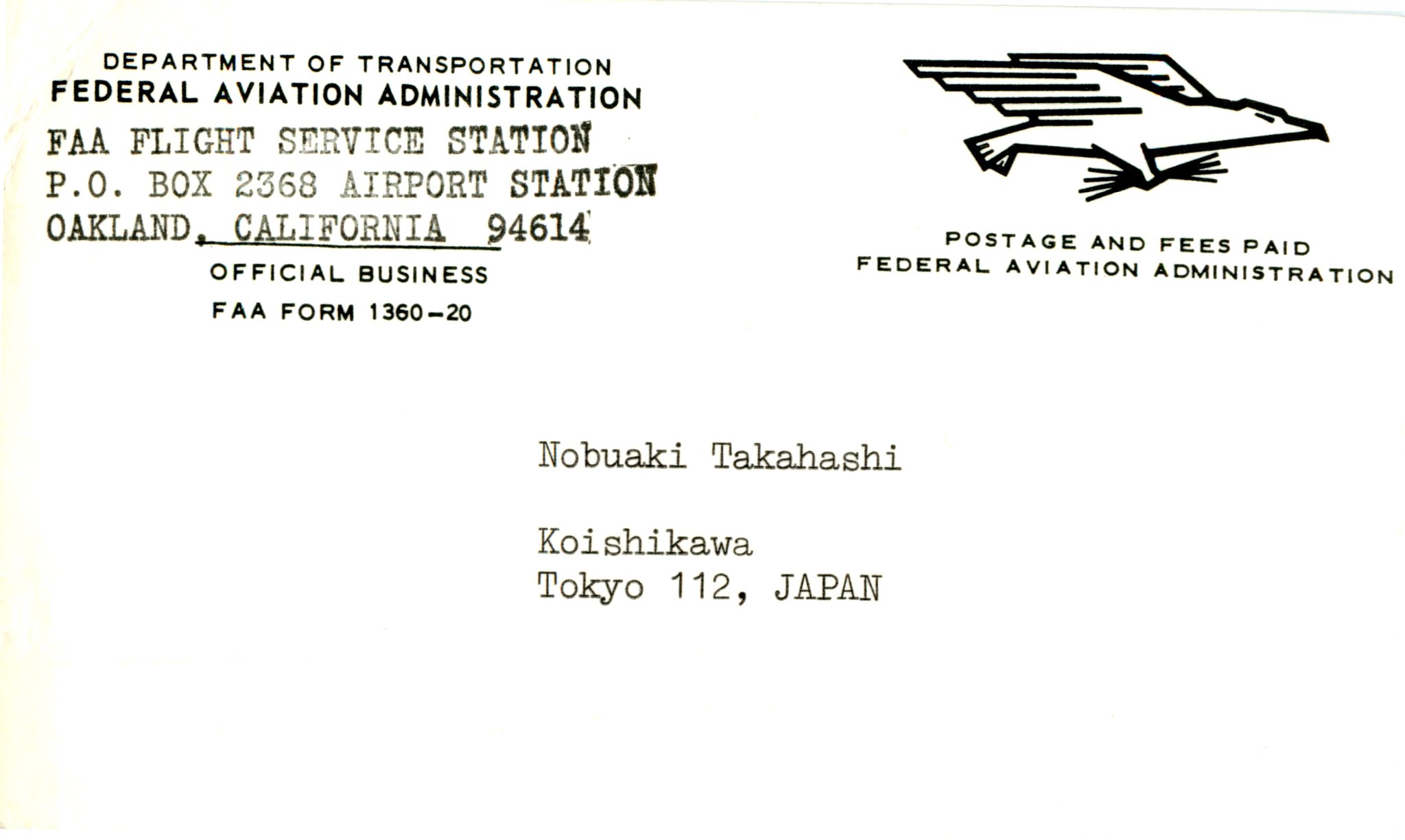This image is an older black-and-white postcard in landscape orientation, resembling the front of a mailed letter. The postcard's upper right-hand corner features a meticulously drawn black-lined eagle clutching items in its claw, facing right. Below the eagle is the text, "Postage and Fees Paid, Federal Aviation Administration." The upper left-hand corner bears a return address stamped for the "Department of Transportation, Federal Aviation Administration, FAA Flight Service Station, PO Box 2368, Airport Station, Oakland, California, 94614," with "California" underlined. Directly underneath this stamp, it reads, "Official Business, FAA Form 1360-20." The central portion of the postcard contains a typed address made with a typewriter, which reads, "Nobuaki Takahashi, Koishikawa, Tokyo 112, Japan." The postcard also exhibits signs of wear, including a faint gray line across the top, a pinkish area, and a slightly crumpled upper corner along the side.